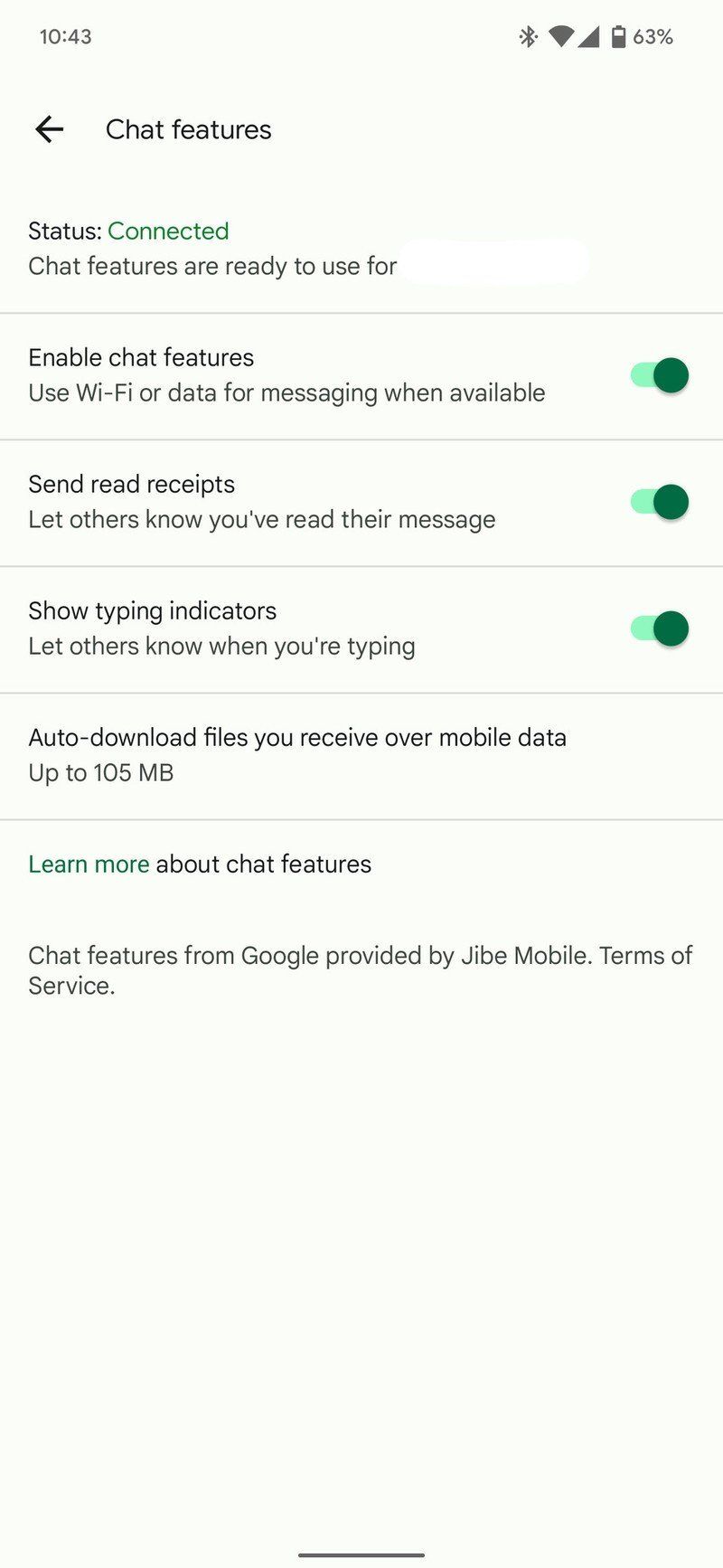Screenshot of a cell phone displaying chat features settings.

The screenshot shows the settings interface of a cell phone with a white background and black text. At the top left, the time is displayed as 10:43, while on the top right, battery and Wi-Fi icons indicate the phone's status.

Below the status bar, the text "Chat Features" with a leftward arrow is visible, indicating a back navigation option. Beneath that, there is a line of small text starting with "Status: Connected" in green, signifying that the chat features are active.

The main content of the screen includes several toggle switches with explanations:
1. "Enable chat features" - Allows the use of Wi-Fi or data for messaging when available, and the green slider indicates it is turned on.
2. "Send read receipts" - This feature lets others know when you have read their messages; it is also toggled on with a green switch.
3. "Show typing indicators" - Displays to others when you are typing a message, which is enabled as indicated by the green switch.
4. "Auto-download files" - Automatically downloads files received over mobile data up to 105 MB.

At the bottom of the screenshot, there is a link labeled "Learn more about chat features," followed by some legal text stating "Chat features from Google provided by Jibe Mobile, Terms of Service."